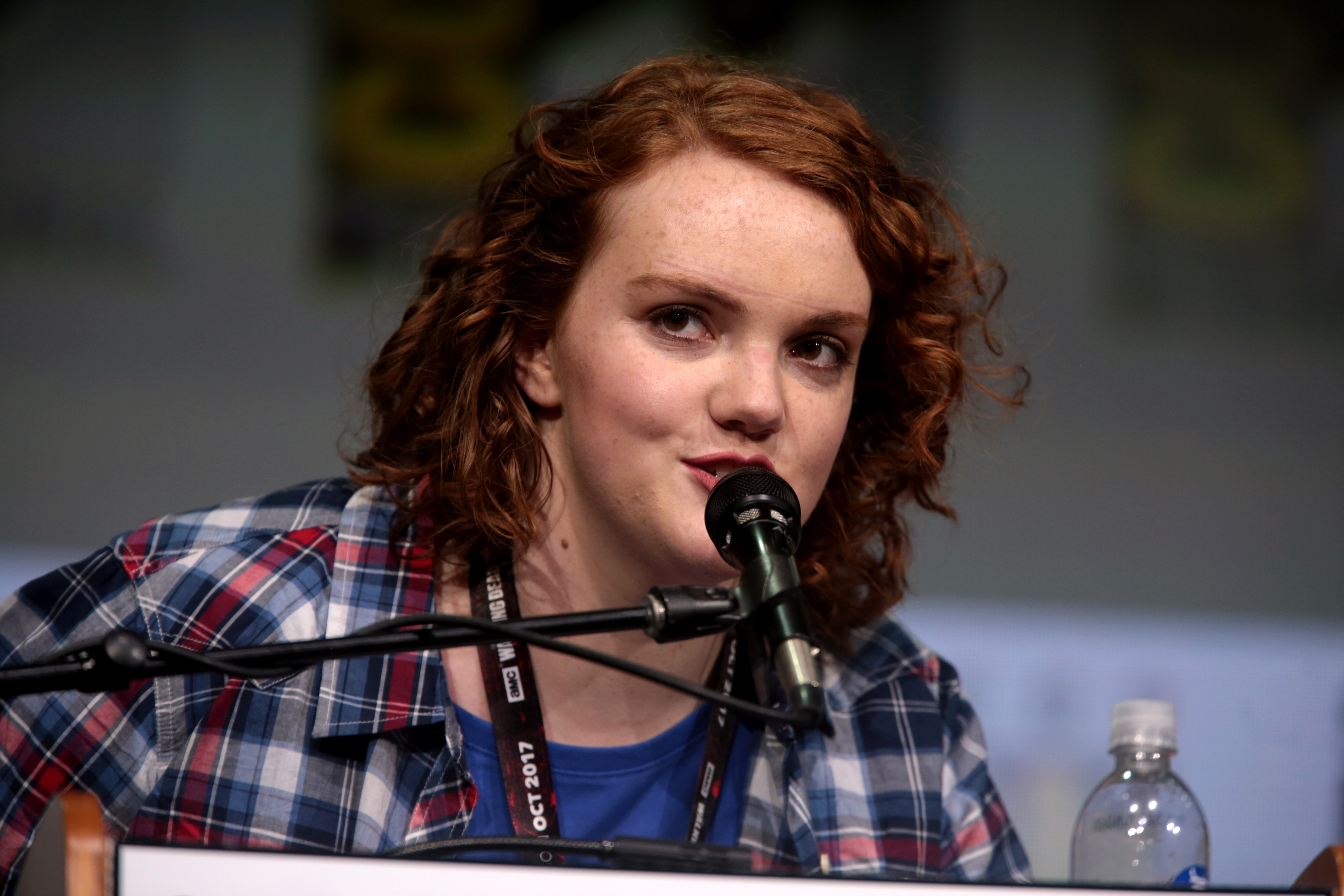In this wide rectangular photograph, an actress with short, curly red hair and pale, freckled skin is speaking into a mostly black microphone at Comic-Con in San Diego. Captured from the shoulders up, she gazes toward the top left corner of the image. She wears a blue t-shirt layered underneath a plaid flannel shirt that features colors like dark blue, gray, white, red, light blue, and black, complete with a collar. A black lanyard hangs around her neck. In front of her, on the table's edge, sits a bottle of Smartwater with a visible blue logo and a clear cap. The microphone, mounted on a stand, extends horizontally with a black wire wrapped around it. Her red eyebrows frame her brown eyes, adding to her distinct appearance as she engages with the audience.